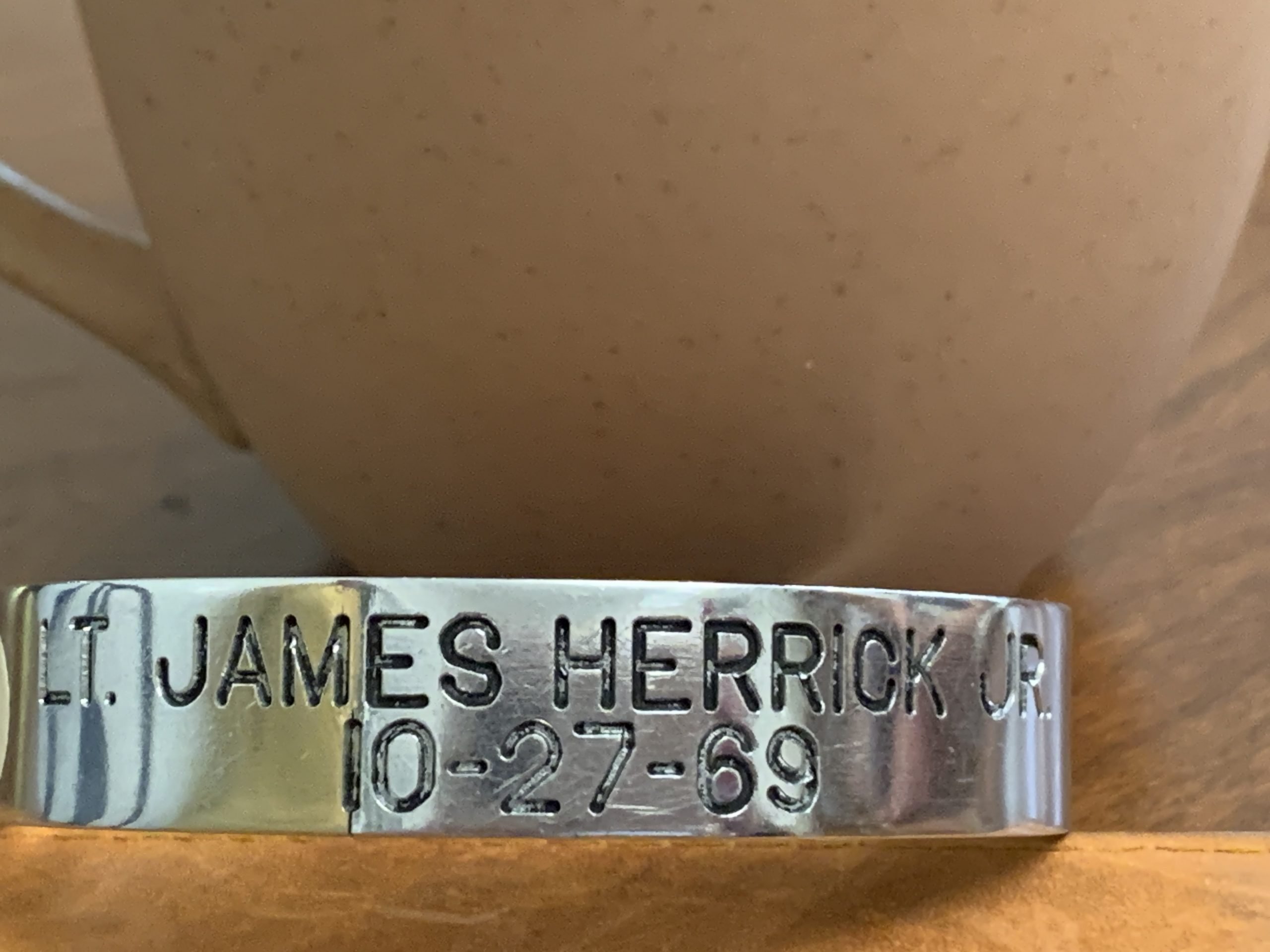The image portrays a close-up of a silver bracelet engraved with the name "Lt. James Herrick Jr." and the date "10-27-69," likely indicating a birthdate. The bracelet lies flat on a brown wooden table. In the background, a cream-colored coffee mug is visible, contributing to the homey and informal setting. A whitish-gray rounded ceiling is also faintly visible, providing slight contextual detail to the room. The bracelet appears to be the focal point, with the coffee mug subtly placed behind, enhancing the overall composition of the scene.